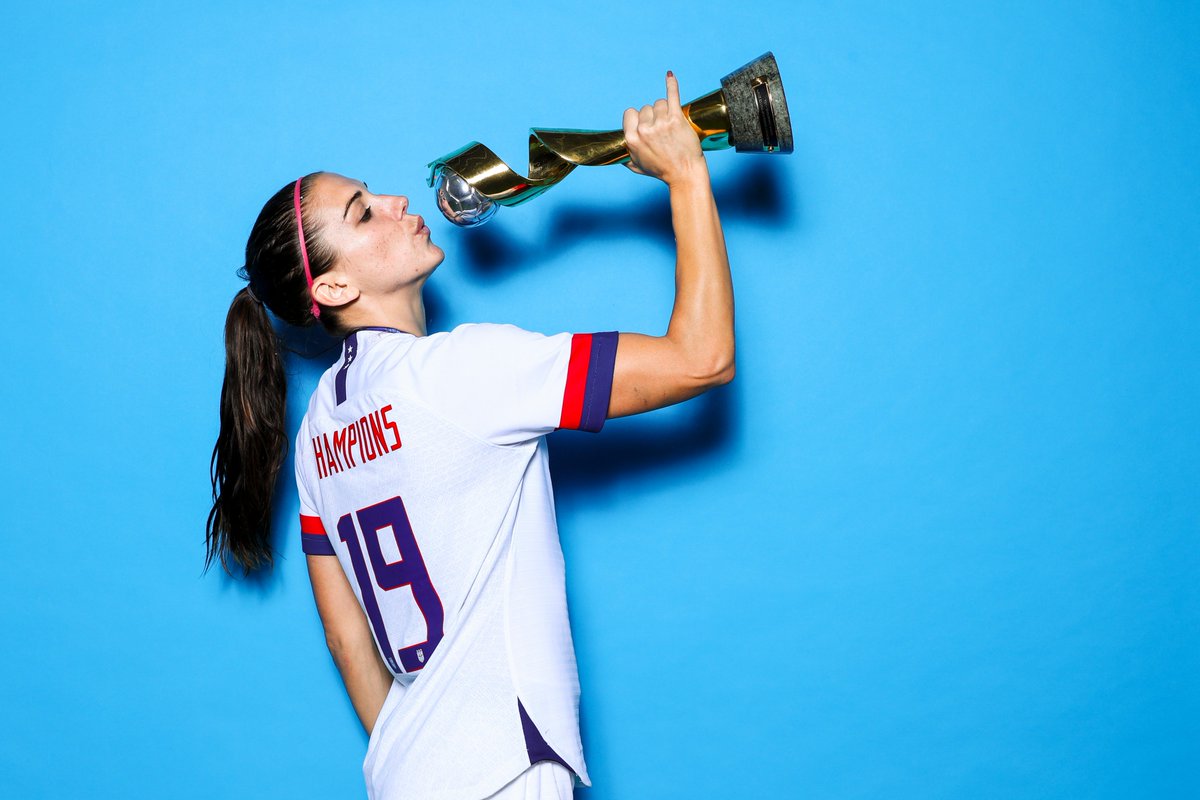In this vibrant color photograph, a jubilant female volleyball player is captured celebrating her victory. She stands against a blue backdrop, proudly displaying a trophy. The athlete has long dark hair pulled back into a ponytail, secured with a red headband that keeps stray hairs in place. She is dressed in a white volleyball uniform, featuring a white jersey with the number 19 in bold blue lettering on the back and "Champions" written in red, although the letter 'C' is obscured. Her sleeves are accented with red and blue stripes. With her right hand, she is holding up a trophy, which is topped with a volleyball, in a dynamic pose that appears as if she is theatrically blowing on it, evoking a sense of triumph and celebration.